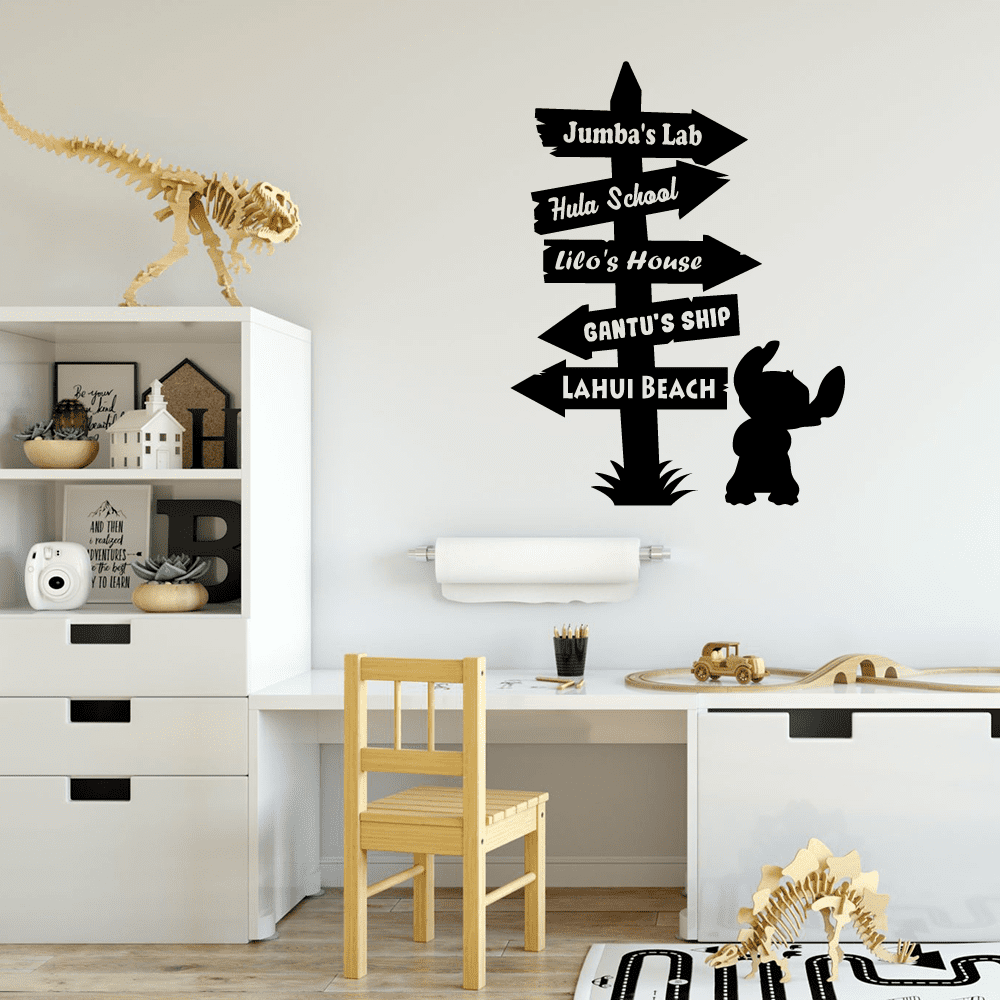This square picture captures what appears to be a child's bedroom, dominated by shades of white and light brown, with notable black accents. The walls are painted white and prominently feature a whimsical black directional sign, which indicates various locations from the "Lilo and Stitch" universe, such as "Jumba's Lab," "Hula School," "Lilo's House," "Gantu's Ship," and "LaHui Beach," each pointing in different directions. To the right of this sign, there's a small black outline resembling a gremlin or troll profile. A roll of paper towels hangs below the sign.

On the left side of the room, a white shelf unit with three drawers at the bottom and two open shelves sits against the wall. The shelves hold various knickknacks, including a white Polaroid camera and a tan, skeletal dinosaur model perched on top.

A low-set desk, coupled with a matching brown wooden chair, is situated on the right side. On the desk, there are wooden car tracks and another tan skeletal dinosaur is strewn on the textured brown tile floor, which mimics the appearance of wood. The overall ambiance is both playful and organized, capturing the essence of a child's imaginative space.